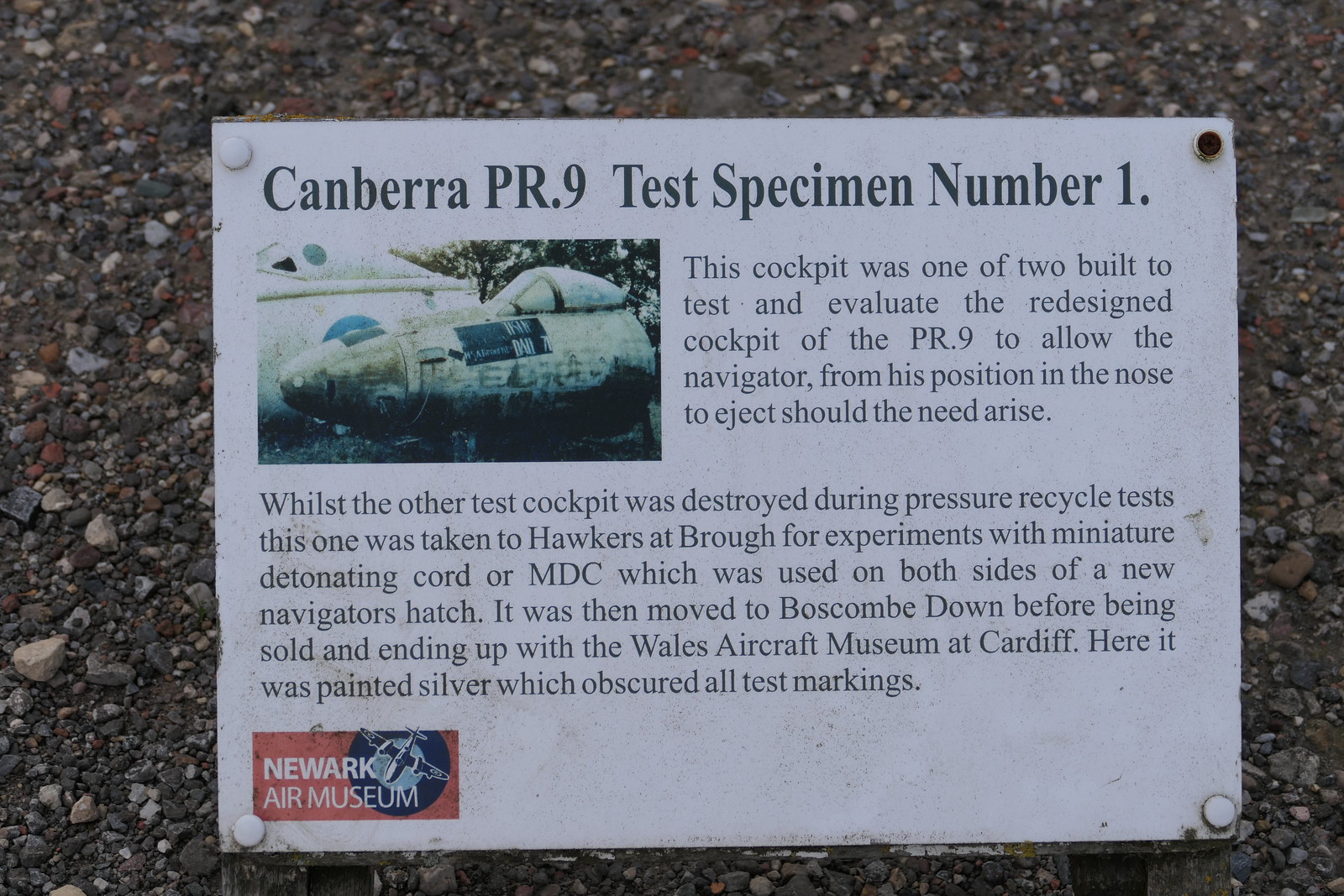Mounted on a granite wall composed of variously colored small rocks and secured with white studs, this metallic, predominantly white placard details the Canberra PR.9 test specimen number one. At the top, the black text reads: "Canberra PR.9 test specimen number one." Below and slightly to the left is an image of a cockpit, accompanied by text that reads: "This cockpit was one of two built to test and evaluate the redesigned cockpit of the PR.9 to allow the navigator from his position in the nose to eject should the need arise." Another column of text below describes the fate of the two test cockpits: "Whilst the other test cockpit was destroyed during pressure recycle tests, this one was taken to Hawkers at BRO for experiments with miniature detonating cord (MDC), which was used on both sides of a new navigator's hatch. It was then moved to Boscombe Down before being sold and ending up with the Wales Aircraft Museum at Cardiff. Here it was painted silver which obscured all test markings." Finally, in the bottom left corner is a small, red rectangle containing a blue image of a cockpit, labeled "Newark Air Museum" in white letters.